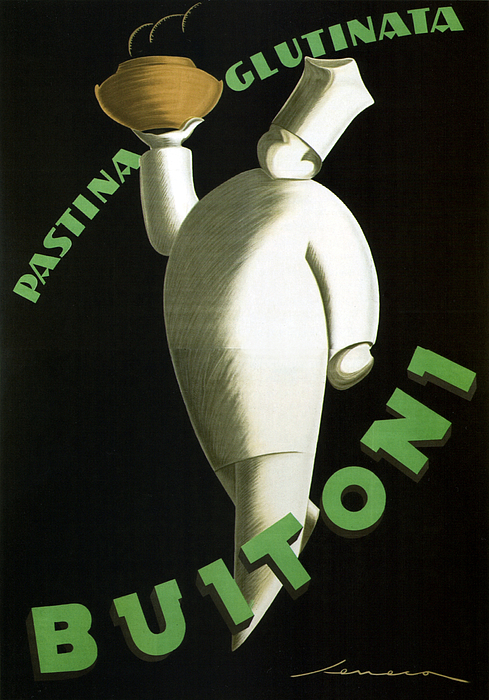This digital artwork features a stylized advertisement set against a black background, depicting a large, white chef figure in the center. The chef, with an exaggeratedly tall hat and minimal facial features, is facing left while holding a steaming, large brown bowl aloft in his right hand. The steam rising from the bowl hints that it contains something hot, likely pasta. The figure blends from white on the right to brown and gray shading on the left, suggesting a hand-drawn pencil technique rather than computer rendering. The bowl is colored in shades of yellow to orange gold. There is text in the image that says "Pastina Glutenata Buitoni," suggesting a gluten-free pasta by the Italian manufacturer Buitoni. Additionally, there is an artist's signature in the bottom right corner, though it is not clearly legible. Overall, the piece combines the whimsical design of the chef with the professional look of a vintage advertisement.